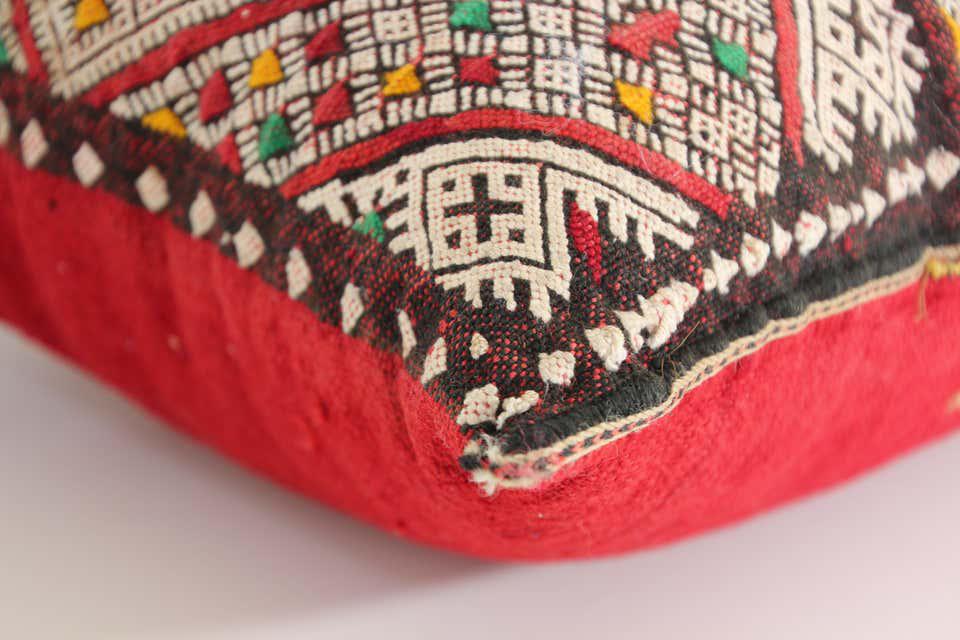This image is a detailed, close-up color photograph of a pillow cover, presented in landscape orientation. The bottom section of the pillow is a deep red, while the top section features a vibrant, intricate Aztec-inspired design. This design is elaborately embroidered with distinctive elements such as rows of black and white brick patterns, interspersed with vivid yellow, red, and green stitching. Prominent within the design are white chain stitches, resembling a mixture of geometric shapes like triangles and stars. These white stitches are highlighted by contrasting red, black, and yellow threads. The pillow’s border is defined by a blackish-gray trim adorned with cream-colored diamond stitches and red threads, suggesting a detailed finish. The photograph captures only a portion of the pillow, approximately a quarter, focusing on the upper arc of the fabric where the detailed stitching is most prominent. The background, a light gray, provides a neutral backdrop that accentuates the rich, colorful patterns of the pillow, conveying a sense of photographic representational realism.